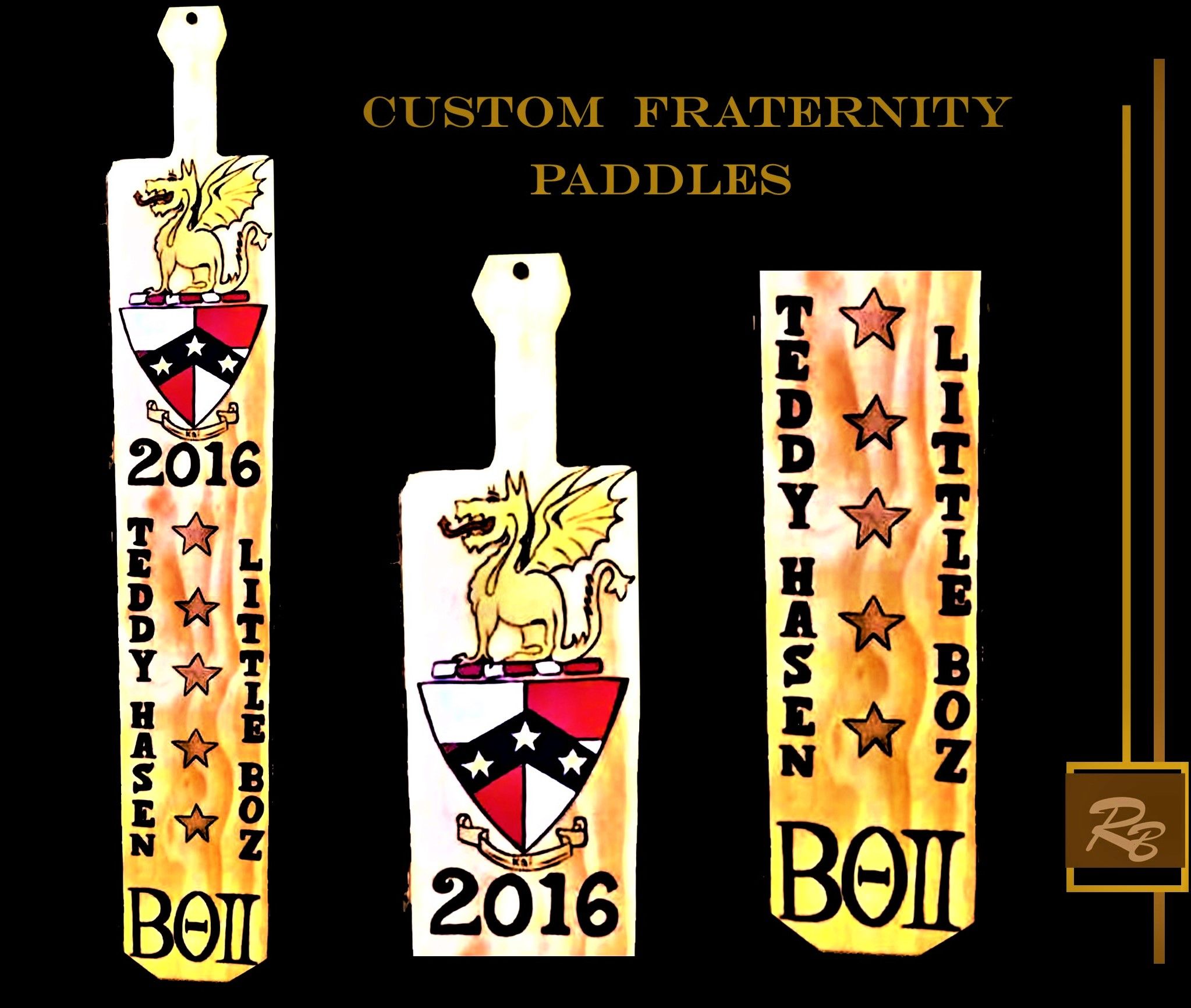The image displays a collection of three custom fraternity paddles set against a black background. The largest paddle, positioned on the left, features the inscriptions "2016," "Teddy," "Passion," and is adorned with little bows. The center paddle, marked "2016," is distinguished by a dragon perched atop a flag. On the far right, another paddle bears the words "Teddy," "Passion," and is similarly decorated with little bows. Above the paddles, the phrase "Custom Fraternity Paddles" is prominently displayed. The paddles showcase a rich palette of intricate colors, including hues of brown, gold, red, white, silver, yellow, and pale yellow, contributing to the detailed craftsmanship of the designs.